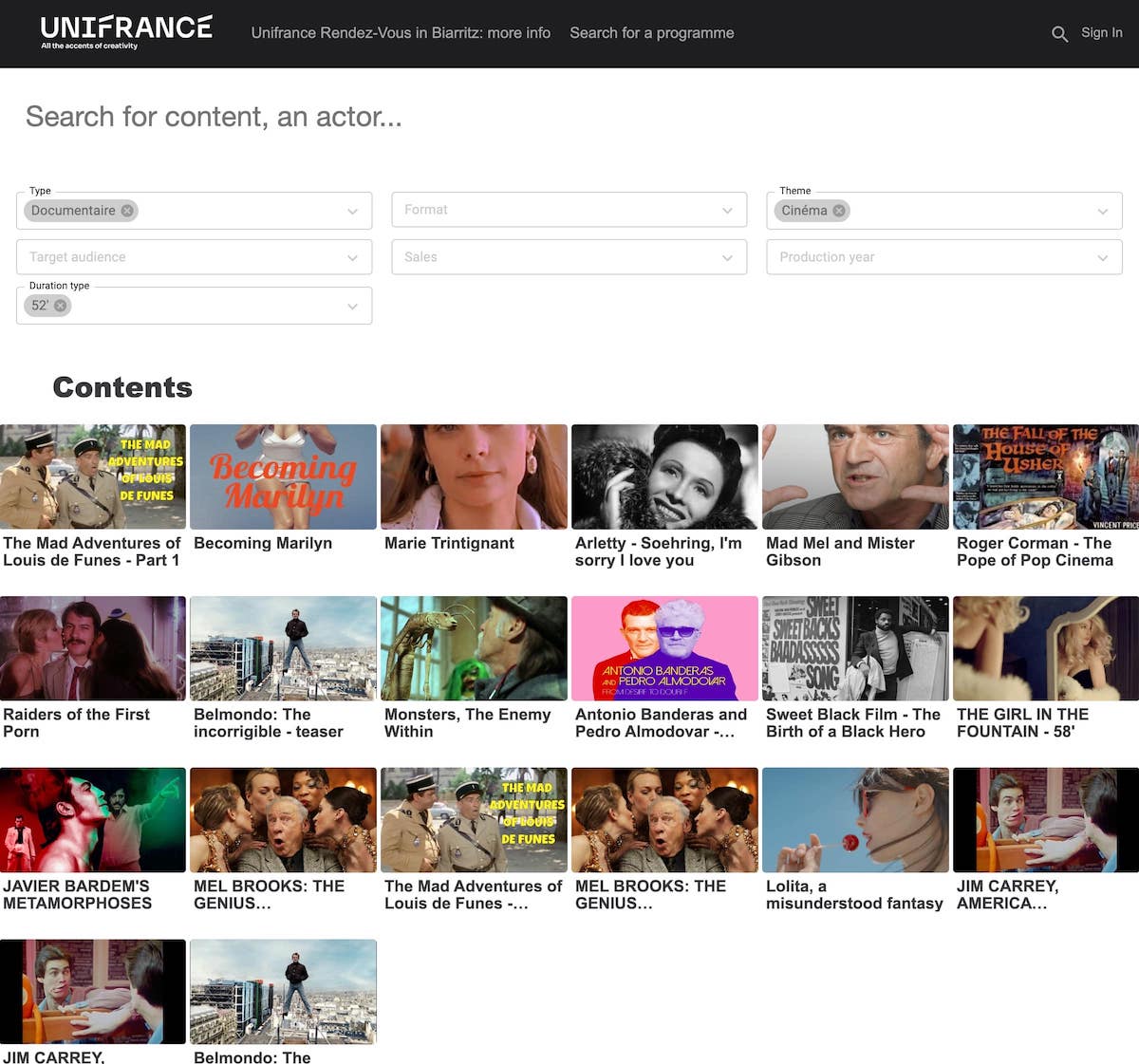**Detailed Caption:**

The image depicts a web page from the Unifrance website, characterized by a white background with a logo positioned at the top reading "Unifrance" with stylized accent marks. Along the right-hand side, navigational options such as "Rendezvous," and "Sign In" are clearly visible. Below the Unifrance header, there is a prominent search bar inviting users to 'search for content and actors.'

The interface includes several interactive fields: 
- A "Type" dropdown menu currently showing a category of "Documentary."
- An unclear "Target Audience" field that is grayed out.
- A "Duration" field that stands at "52 minutes."

Further to the right, additional dropdown menus include:
- A grayed-out "Format" field pertaining to sales details.
- A "Theme" field, which is set to "Cinema" (focusing on movies).
- A "Production Year" selector.

In the main content area beneath these fields, bold lettering spells out "Contents," organizing the cinematic offerings into rows and columns. Specifically, three full rows contain six movies each, with a partial fourth row listing two films. 

Highlighted movie titles include:
- "The Mad Adventure of Louis de Funès, Part One"
- "Becoming Marilyn"
- "Mel Gibson's Raiders of the First Horn"
- Other lesser-known titles resembling B-rated movies.

The layout and options suggest a user-friendly platform dedicated to exploring a variety of films, emphasizing international cinema selections.